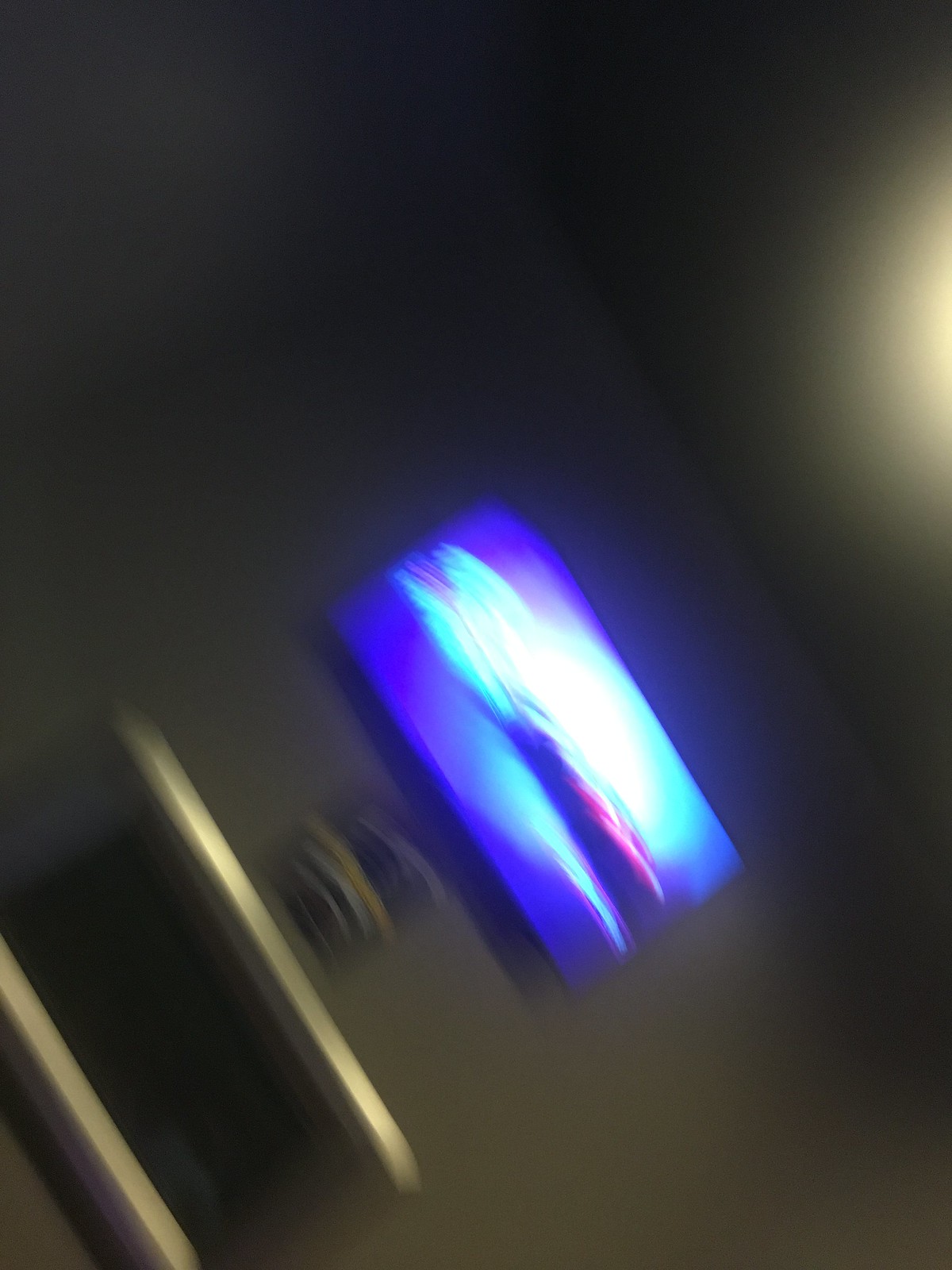This photograph, taken at an off-angle and in portrait mode, presents a diagonally tilted, out-of-focus composition with a blurred haze permeating the entire image, making detailed identification challenging. The scene is set against a dark gray to almost black background, including both the wall and the ceiling. In the upper right corner, a bright light source casts a soft glow, contributing some gray tones to the surroundings. Dominating the central area of the image is a glowing rectangular object, likely a television screen, displaying streaky, blurred swirls of purple, light blue, pink, and magenta. Below the screen are two thin, silver shelves, and there is an indistinct, black-and-yellow square shape adjacent to them. The entire photograph captures an enigmatic and abstract ambiance due to its severe blur and diagonal orientation.